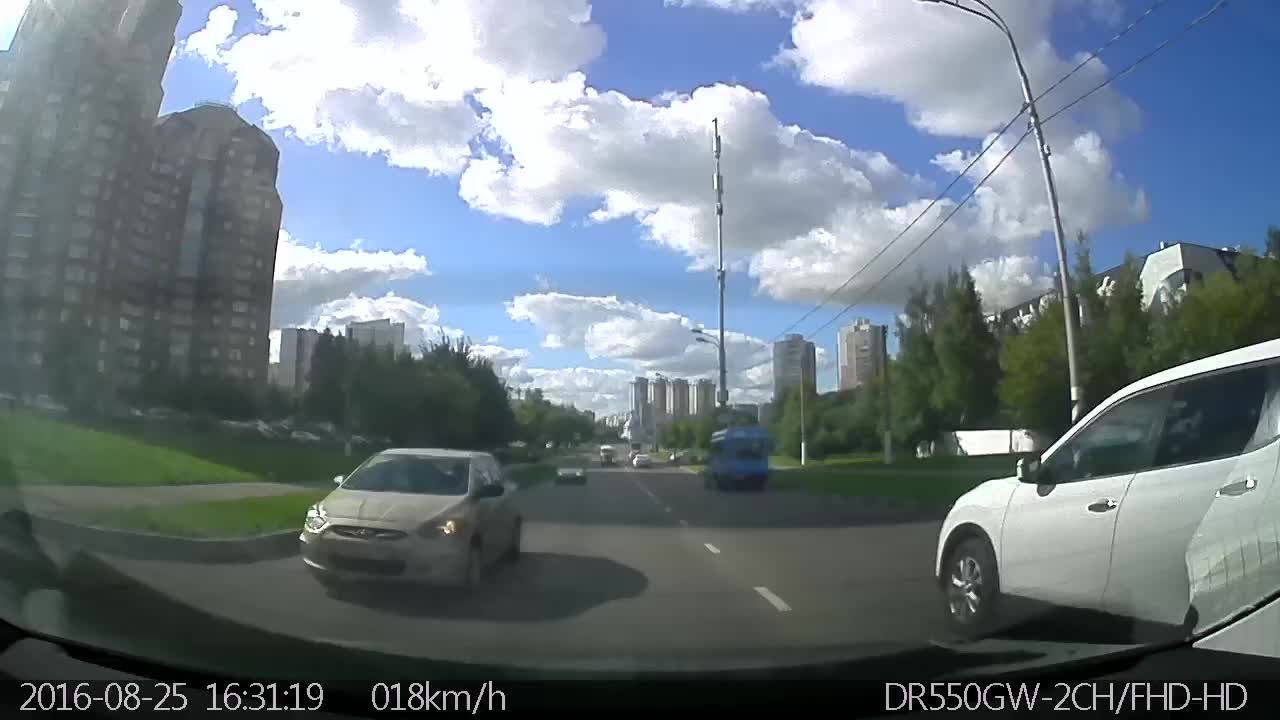The image appears to be a photograph taken from a dash cam, potentially mounted on either the front windshield or back window of a car. The image is dated August 25, 2016, at around 4:31 PM, as indicated by the timestamp "2016-08-25 16:31:19" in the bottom left corner. The speed is recorded as 18 kilometers per hour (approximately 11 miles per hour). The bottom right corner features a serial code "DR550GW/FHD-HD."

The scene captures a busy city street with cars, including a white car and a tan car closest to the camera, and a blue bus in the background. Surrounding the street are green shrubbery, grass, and tall high-rise apartment buildings interspersed along the horizon. The sky is a light blue with large, puffy clouds, suggesting a clear day. Utility poles and trees are also visible, adding to the urban landscape. The photograph's setting has elements that could suggest cities like Toronto or Denver, noted for their close-to-ground clouds and combination of urban and natural features.